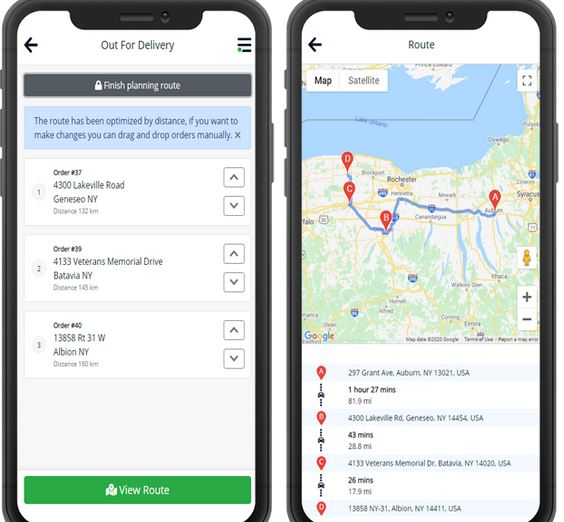The image depicts two smartphones placed side by side in a square-ish frame. Both phones appear to be identical, each enclosed in a black case, with the top and bottom portions slightly cropped out of the image. The left phone displays a delivery management interface with a white background. At the top, it indicates "Out for Delivery" alongside a wide gray rectangle stating "Finish Planning Route." Below, a blue rectangle provides instructions, "The route has been optimized by distance. If you want to make changes, you can drag and drop orders manually," followed by three order numbers with corresponding addresses.

The right phone screen shows a map application, presumably Google Maps, labeled "Route" at the top. The map highlights four points marked as A, B, C, and D, likely corresponding to the delivery addresses listed on the left phone. The visible map area includes locations such as Rochester and Syracuse, suggesting that the image pertains to a delivery route in northern New York State.